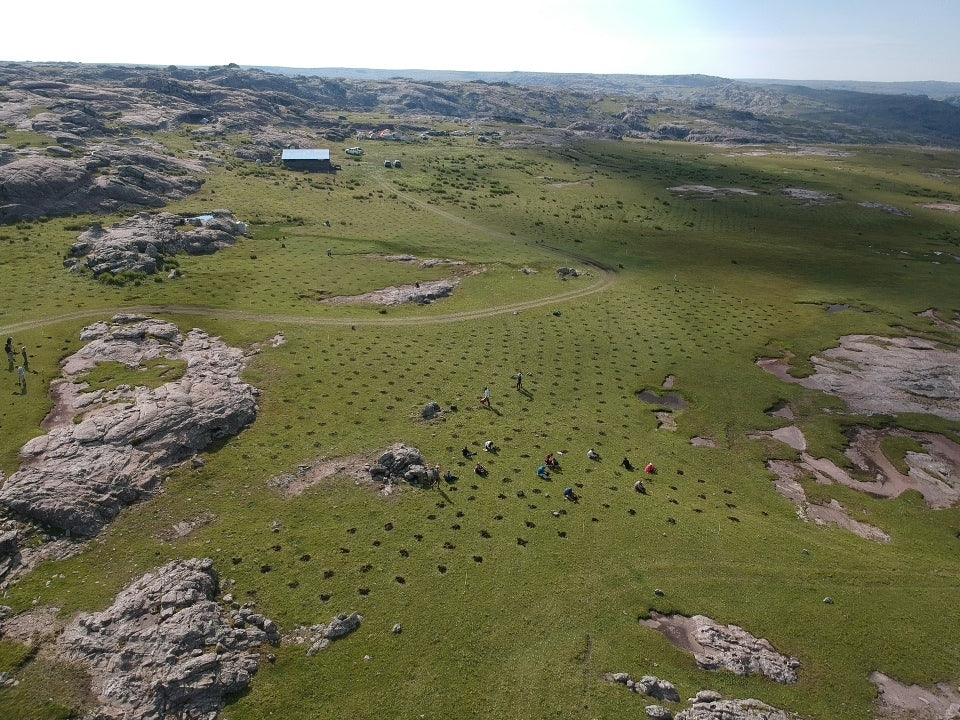This aerial photograph captures a vast, flat grassy field sliced by numerous holes that create a dotted pattern stretching from left to right across the terrain. The grassy expanse is punctuated by large rock formations that rise prominently from the ground, especially noticeable on the left side. Scattered throughout the field are people engaged in an indistinct activity – possibly planting or digging – some of whom are distinguishable by their colorful shirts in hues of orange and blue. The background reveals a mountainous landscape which adds depth to the scene, and a modest structure with a brown facade and silver tin roof, potentially a house or barn, stands quietly amidst the greenery. The overall composition is bathed in a soft light, possibly from a setting or rising sun, casting a serene glow over the field despite the subdued and muted palette of colors in the image.